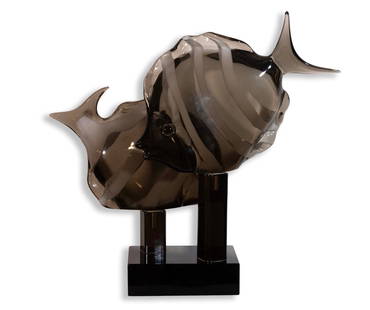This photograph captures an exquisite glass sculpture of two tropical fish, meticulously crafted to resemble flounders with their rounded bodies and elegant form. Both fish, rendered in dark black, translucent glass with grayish hues, are artfully arranged on a glossy black stand, exuding a luxurious, polished finish that hints at marble or metal. The stand, composed of two distinct legs or pillars—one noticeably shorter than the other—supports the fish in a dynamic display, with each fish facing opposite directions as if swimming in a synchronized dance. The taller leg holds a fish diving down, its tail above its head, on the right-hand side, while the shorter leg presents another fish whose head is obscured, contributing to the impression of movement and depth. This intricate piece stands against a stark white background, highlighting its intricate details and the masterful craftsmanship, possibly from hand-blown glass techniques, suggesting its place as a sophisticated artwork fit for a gallery or elegant interior setting.